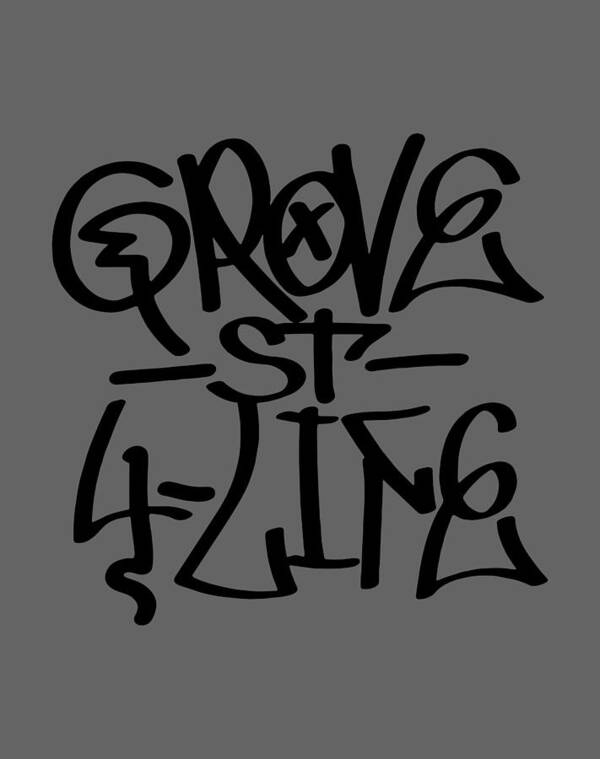The image showcases a gray background that resembles a large, poster-sized rectangle with elaborate graffiti art. Central to the design are thick, black graffiti-style letters that spell out "Grove Street 4 Life." The highly stylized letters feature unique attributes: the 'G' has a zigzag lightning bolt extending from its center, the 'R' appears fairly conventional, the 'O' contains an 'X' in its middle, and the 'E's in both "Grove" and "Life" have a six replacing their upper portions. A dash separates "S-T" which looks normal, and the number '4' has a squiggle reminiscent of an 'S' at its base. The 'F' also has a notably crooked top portion. Overall, the design is exclusively black on a gray background with no additional decorations, bringing a strong, graphic impact through its bold, wavy lines and intricate details.